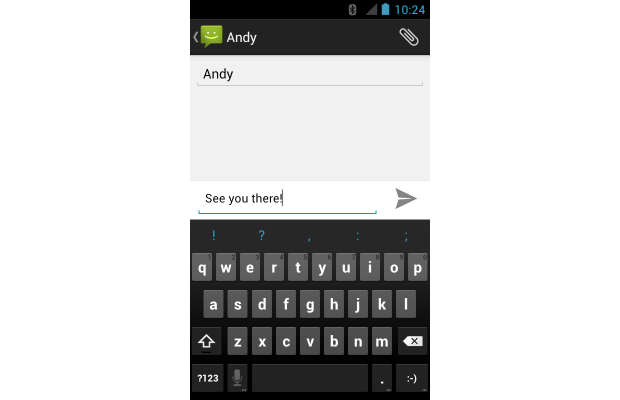This is a detailed screenshot from a cell phone display. At the very top of the screen, the time is displayed as 10:24 in the upper right-hand corner, accompanied by a blue battery icon, a cellular signal icon, and a Bluetooth icon. Below this top bar, on the left side, there is a square speech bubble with two eyes and a smiling mouth on a green background. To the right of this, in white text, the name "Andy" is displayed. On the far right side of this section, there is a paperclip icon angled diagonally to the upper left.

Directly below this section, there is a grey background area featuring a darker grey horizontal line, with the name "Andy" written on the line. Further down, there is a smaller white box that stretches across the page, containing a thin horizontal blue line. Above this blue line, the text "See You There" is displayed, with a right-facing arrow on the far right edge of the box. Beneath this, the screen transitions to a dark grey background showing the cell phone's keyboard interface, indicating it is ready for further input.